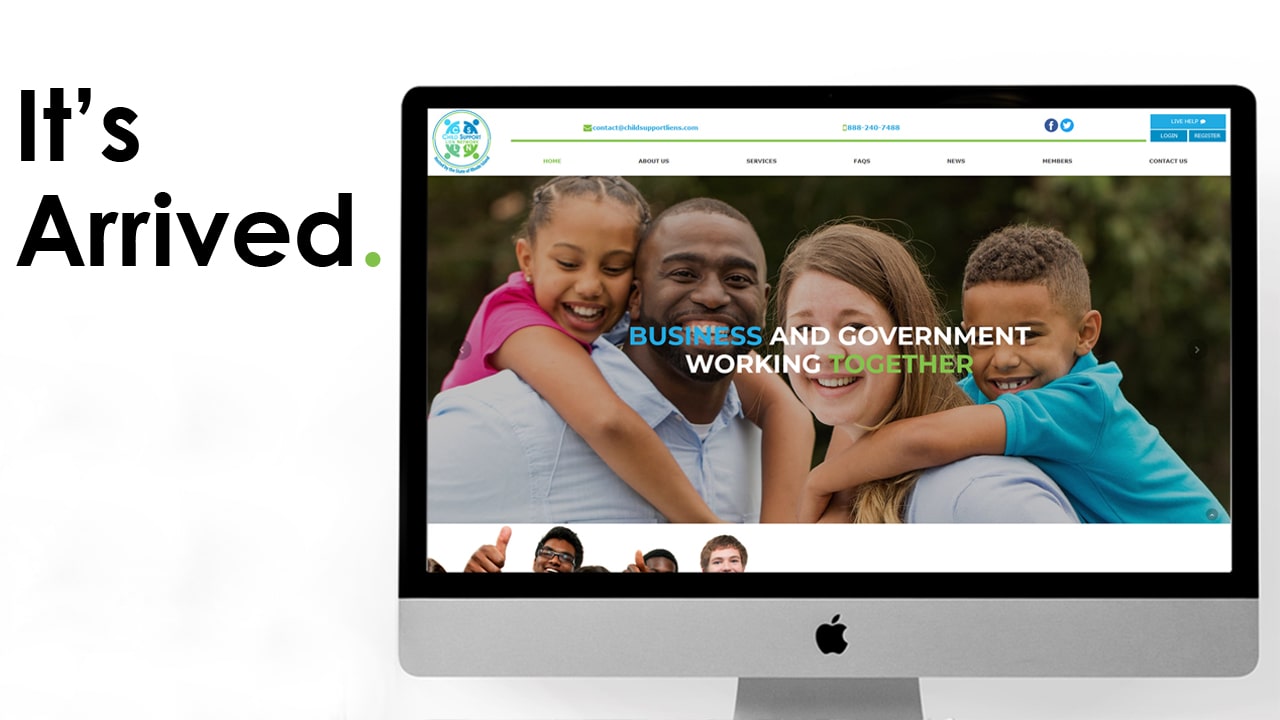This image features a Mac desktop monitor that showcases a sleek two-tone design of gray and black. Prominently placed in the bottom center of the monitor is the iconic black Apple logo. On the screen, a web page is displayed, with a green and blue colored logo situated in the top left corner.

The top of the monitor is lined with various tabs, and in the top right corner, recognizable Facebook and Twitter icons are present. The central part of the screen displays a heartwarming photo of a family: a man and a woman giving piggyback rides to their children. The daughter is joyfully perched on the man’s back, while the son is riding on the woman’s.

Above this image is the text "Business and government working together." On the left side of the screen, the text "It's arrived" is visible, accented with a green dot.